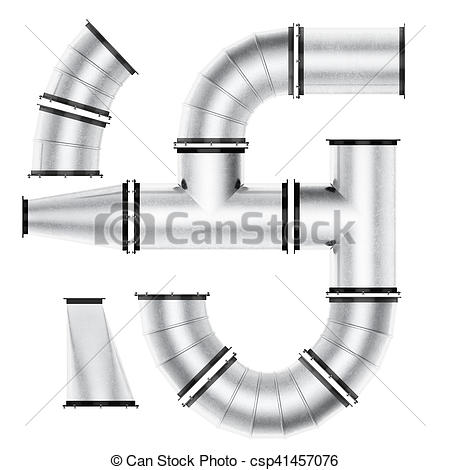The image depicts a complex arrangement of silver metal pipes with prominent black rings at various junctions and ends. These rings sometimes feature white centers. The pipes form an intricate, serpentine pattern, weaving up and down without an immediately discernible organization or direction, incorporating shapes reminiscent of "S" curves and rectangular sections. The background is predominantly white with four muted, light gray dashes forming an X shape. Superimposed at the center is a gray watermark of a camera icon accompanied by the word "Canstock." Below the image is the text "© Canstock Photo CSP41457076" in black.